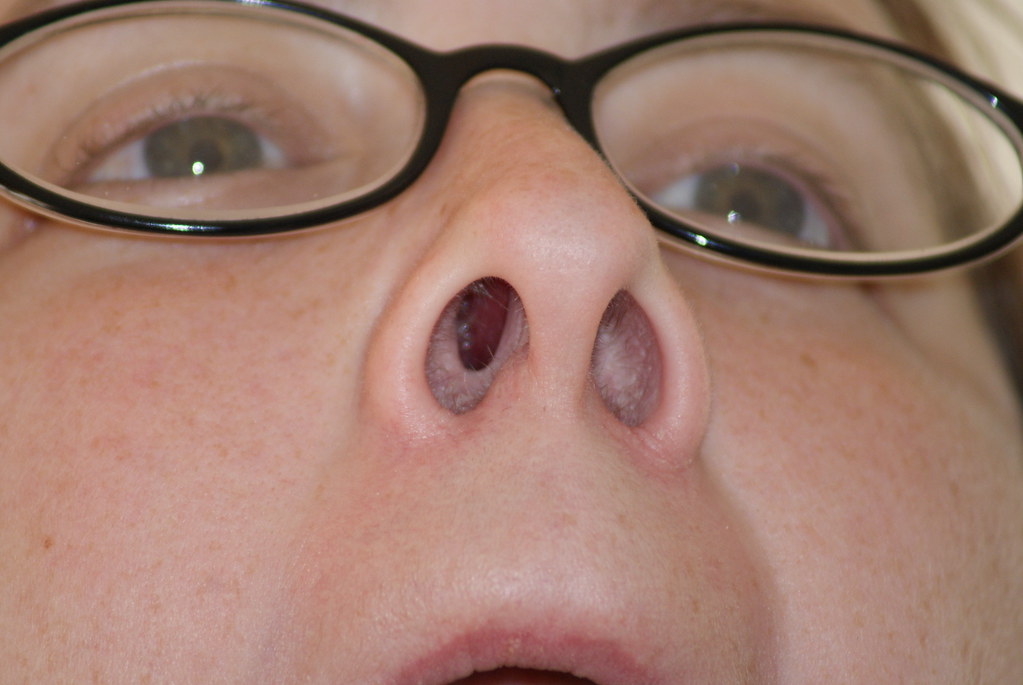This close-up photograph focuses on the midsection of a white woman's face from her glasses down to just below her top lip, captured from a low angle that emphasizes her nostrils. Her pudgy cheeks and fair, freckled skin are clearly visible. She wears round, black-rimmed glasses framing her green or hazel eyes, gazing downwards. Peeking from the top right corner is a glimpse of her dirty blonde hair. The image starkly highlights her open nostrils and nose hairs, making them the predominant feature, with her thin top lip slightly curled. No makeup is visible on her face. The perspective and framing render the photograph particularly unflattering and uncomfortable.